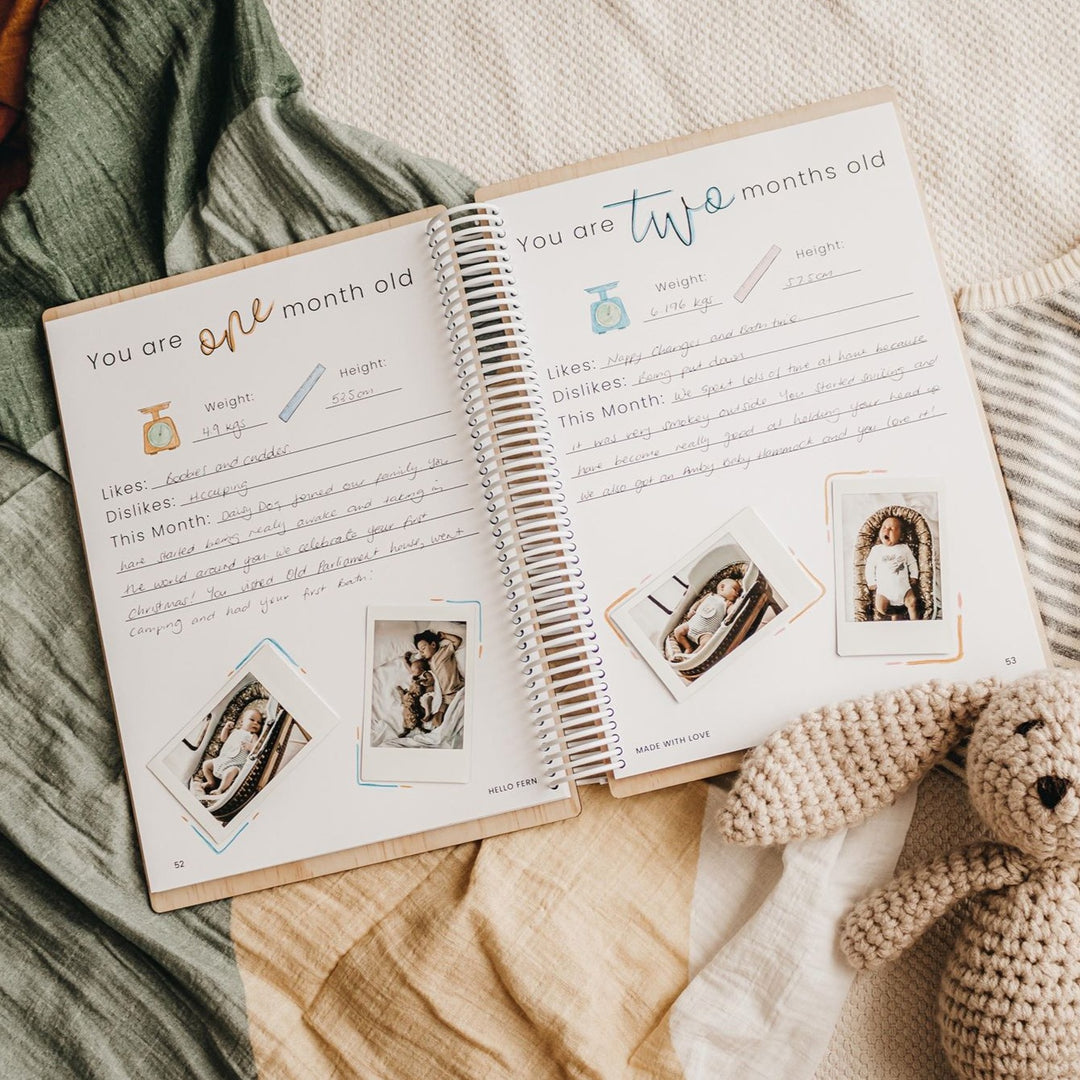This image showcases an open baby memory book resting on a colorful assortment of blankets with neutral and earthy tones such as tan, gray, white, yellow, green, and brown. The book, colored white and beige with a white spiral binding, is open to pages that are titled "You are one month old" and "You are two months old." Each page contains spaces to document the baby's weight, height, likes, and dislikes, along with notes about the month. The entries, written in difficult-to-read handwriting, specify a weight of 4.9 kilograms and a height of 52.5 centimeters for the one-month page, noting likes such as "boobies and cuddles" and dislikes like "hiccuping." Small Polaroid photos are attached to the bottom of each page, capturing moments like a baby in a bassinet and a baby yawning. Beside the book, partially overlapping it, is a hand-knitted bunny rabbit toy. The overall scene gives a cozy and intimate glimpse into cherished moments of early parenthood.